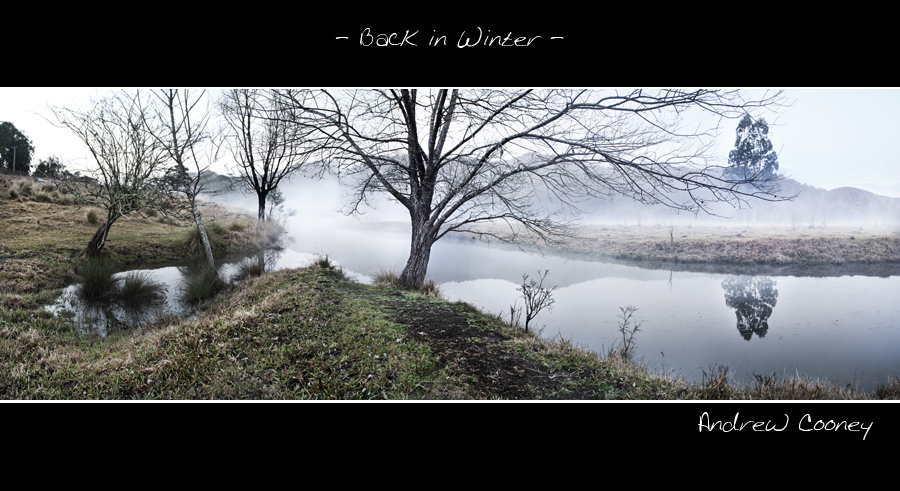This is an outdoor photograph of a calm, reflective stream, possibly a river or creek, framed by narrow black bars at the top and bottom, similar to a widescreen movie. In the top bar, centered in white text, it reads "Back in Winter," while the bottom right corner of the lower bar states "Andrew Cooney." The left side of the image shows an embankment with grassy areas, dirt, and small, bare trees, suggesting a late fall or winter setting. On the opposite side of the stream in the upper right corner, there is dried-out grass, a tall tree whose reflection is visible in the still water, and some fog. In the far distance, the silhouette of hills or mountain ranges can be faintly seen through the mist, enhancing the serene, cold landscape.